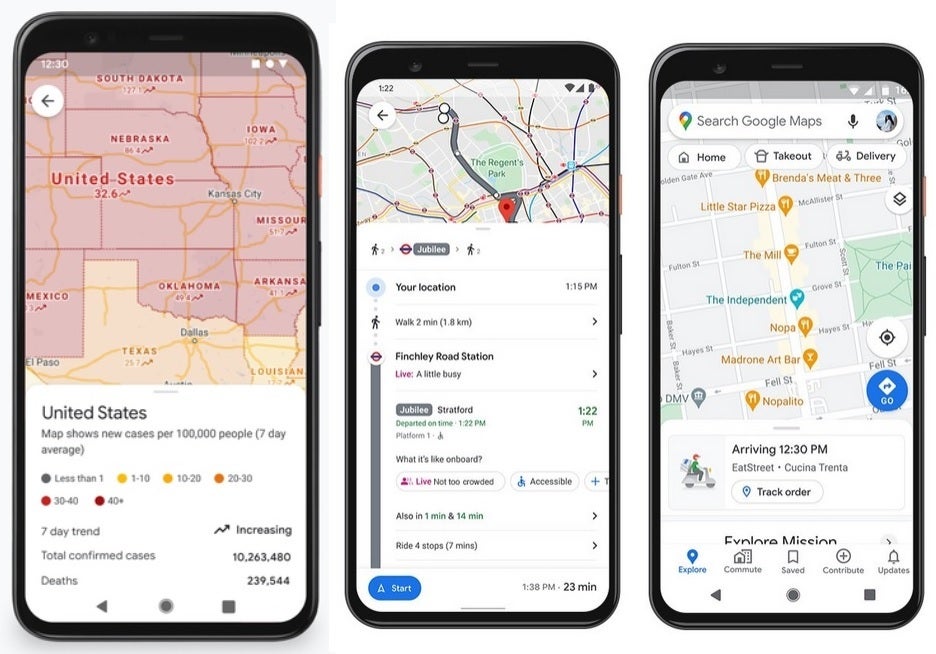The image showcases a row of three smartphones side by side, each displaying a different map and information. The phone on the left is slightly larger than the other two and shows a map of the Central Midwest region of the United States. Below this map, there is a white section indicating “United States” with data on new COVID-19 cases per 100,000 people on a 7-day average. It includes a legend and notes that the 7-day trend is increasing. It also displays a total of 10,263,480 confirmed cases and 239,544 deaths.

The phone in the middle presents a directions map of the Regents Park area. There are small icons indicating walking as the mode of transport, with Jubilee marked as the final destination. At the top of the screen, it shows the user’s location at 1:15 PM, and at the bottom, it states the arrival time at 1:38 PM, a duration of 23 minutes. To the left, there is a blue "Start" button.

The phone on the right screen captures another map, seemingly of a restaurant. It indicates an arrival time at 12:30 PM and includes a "Track order" button for convenience.